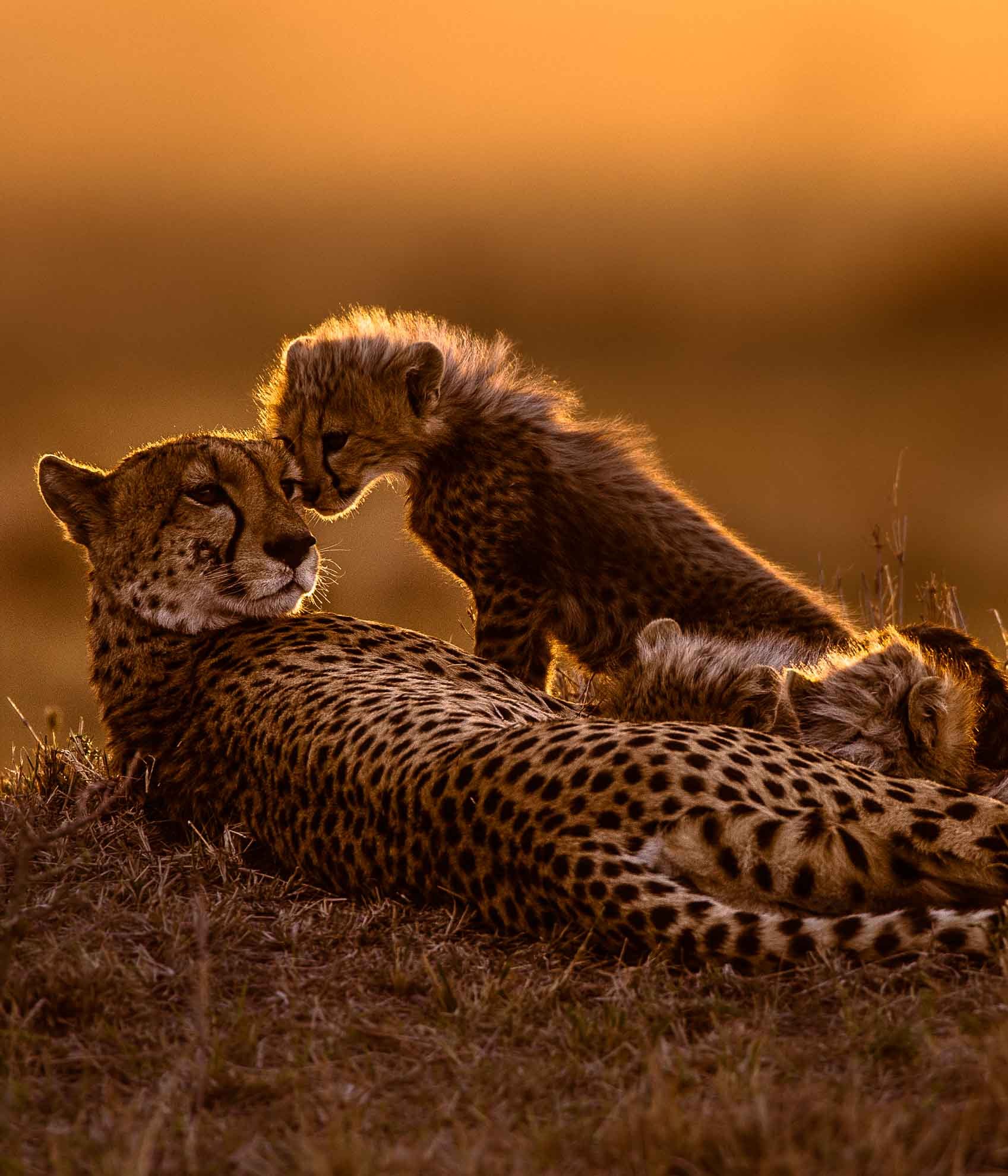This captivating photograph, set against the evocative backdrop of a reddish, honey-gold sunset, showcases the tender bond between a mother cheetah and her cubs in their natural habitat, likely the African savannah. The image is a close-up, vertically oriented, and depicts an adult cheetah, presumably the mother, laying on the dry, tan grass with two visible cheetah cubs. The adult cheetah, with its distinctive black tear marks and spotty coat, gazes towards the right of the frame, her fur glowing warmly in the dim, angled light of the setting sun. 

One cheetah cub, noticeably smaller in size with a petite head, is positioned near the mother’s face, nuzzling affectionately while standing on its hind legs. Another cub, less prominent but discernable, appears to be nursing or cuddling close by. The background is artistically blurred in hues of orange and brown, focusing attention on the finely textured fur and the tranquil scene of familial affection. The cheetahs, all spotted with striking black polka dots, are in a state of peaceful relaxation, depicting a serene moment of wildlife intimacy without any signs of hunting or human presence. The overall atmosphere is bathed in a soft, golden glow, further enriching this exquisite portrait of cheetah family life.